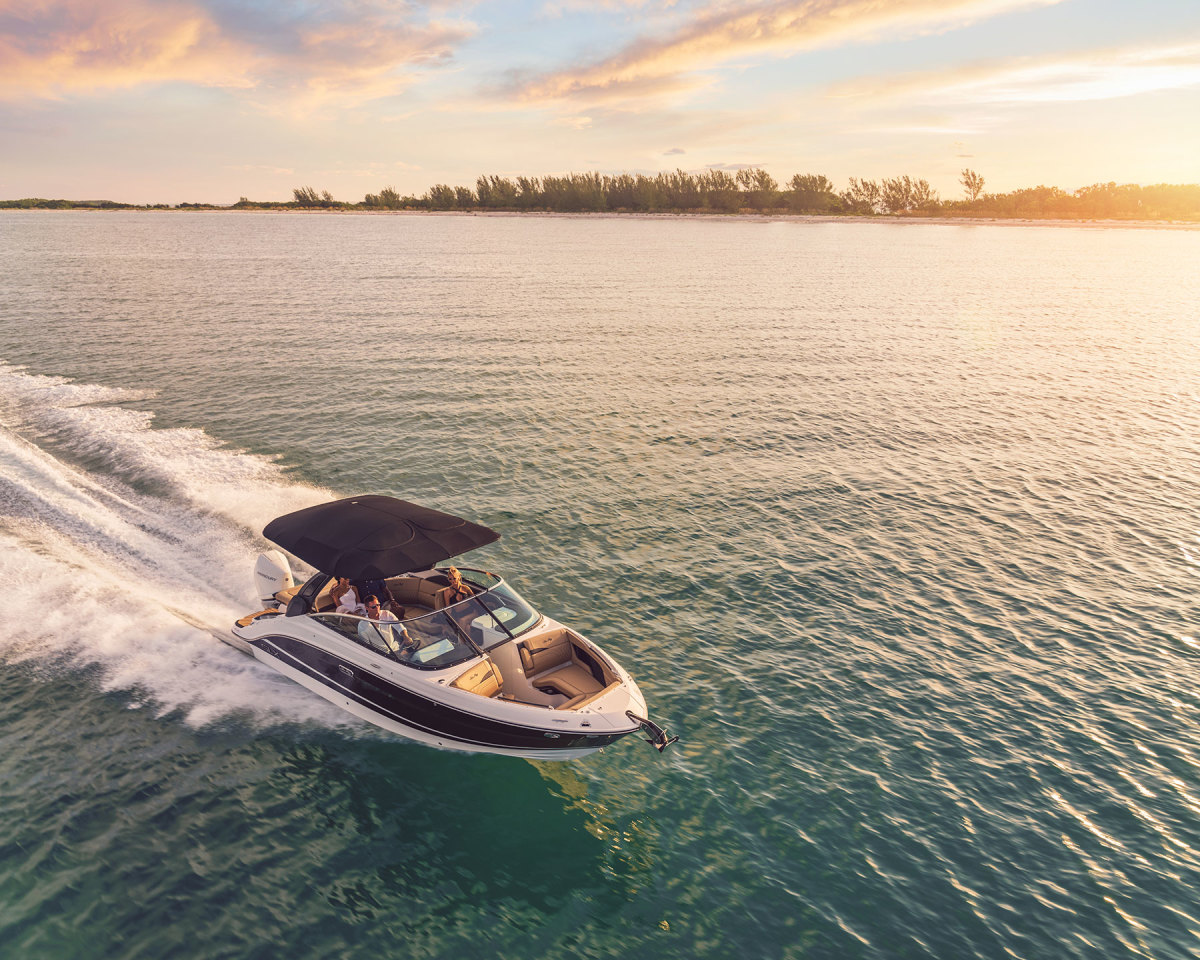An aerial shot captures a small white speedboat with black and brown accents, speeding across a turquoise-blue lake with a foamy white wake trailing behind it. The boat, driven by a man on the right, has a woman in a bikini seated to his left, and possibly another person on board. The open sport boat features a glass windshield, a dark brown canopy top, two seats in front near the bow, and circular seats in the back. The surrounding landscape includes a tree-lined shoreline with a visible cabin and more trees in the distance. The sky is mostly clear with blue hues and puffy white, light blue, and pink-tinged clouds, indicating that the sun is low on the horizon, likely setting. The sunlight casts a gentle glow on the water, adding a serene, almost pastel quality to the scene.